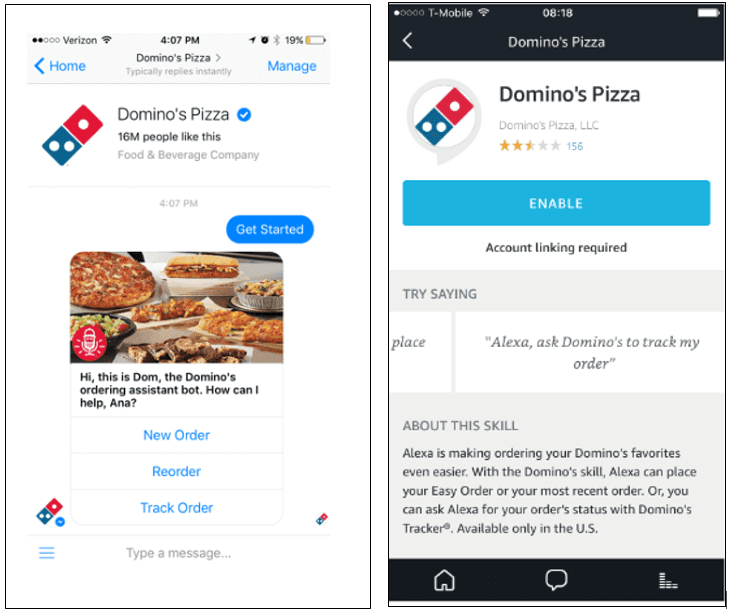The image displays two screens of a cell phone, both showing the Domino's Pizza app interface.

The status bar at the top reveals various indicators: "Verizon," a network with two bars and 5G, Wi-Fi, the time as 4:07 p.m., an alarm icon, Bluetooth, and a 19% battery level, displayed in yellow due to the low charge.

Below the status bar, the interface includes navigation buttons. On the left, a button labeled "Left," a "Home" button highlighted in blue at the center, and a "Manage" button in blue on the right.

Underneath, the app's main interface for Domino's Pizza is visible. It shows that six million people like this food and beverage company. The Domino's logo, a red domino with a single dot and a blue portion with double dots, is prominently displayed. There's a blue circle next to the word "Pizza," featuring a white checkmark inside.

The screen further shows a message timestamped at 4:07 p.m.: "Get started." Below this line, a vibrant photograph of pizzas, sandwiches, and salads is displayed. The message from the Domino's order assistant bot reads: "Hi, this is Dom, the Domino's order assistant bot. How can I help you, Anna? New order, reorder, track order." Underneath this text, there is a field to type a message response.

The second screen provides additional information about the Domino's Pizza app. It shows a rating of 2.5 stars from 156 reviews and mentions that an account link is required to enable certain features. A suggestion is made to use voice commands: "Try saying 'Alexa, ask Domino's to track my order' about this skill." It highlights how the Alexa skill can make ordering Domino's favorites easier by allowing users to place their easy order or most recent order, or check the order status with Domino's tracker, available only in the U.S.